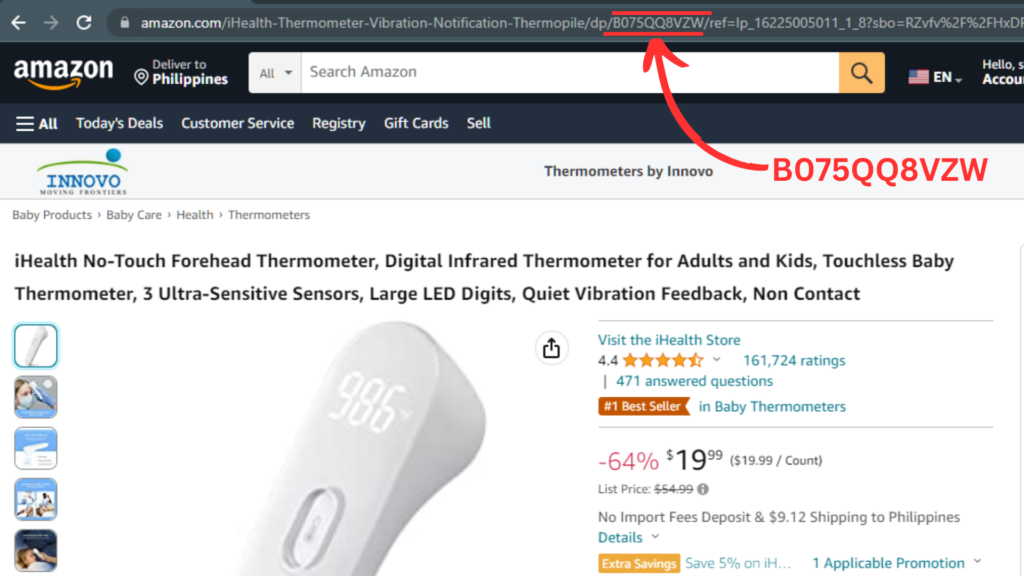The image is a screen capture of a product page on the Amazon.com website, showcasing a "No Touch Forehead Thermometer" designed for both adults and children. The thermometer features digital infrared technology, three ultra-sensitive sensors, large LED digits for easy reading, quiet vibration feedback, and a touchless measurement capability ideal for babies.

At the top of the screen, there is an address field displaying a URL. A specific portion of this URL is highlighted with lines above and below it. Below this, the same number is enlarged and displayed prominently with an arrow pointing upwards towards its original location in the URL. This visual aids in identifying a specific number, likely the order or product number, facilitating users in locating this crucial detail on the Amazon website.